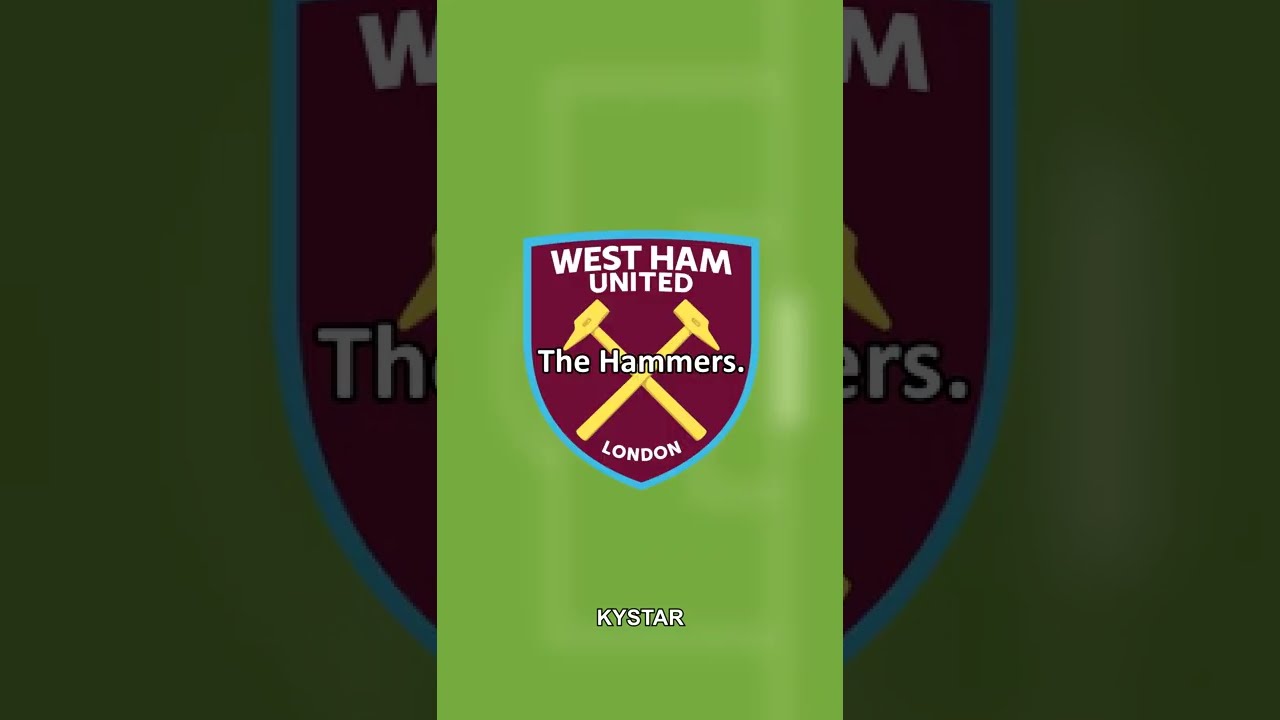This horizontal rectangular image prominently features a central panel with a greenish background that highlights a detailed crest. This crest is colored in maroon and blue, resembling a shield with an insignia at its core. It reads "West Ham United" in white letters at the top, with two golden, crossed hammers centered below the text. Across these hammers, also in white letters, it states "The Hammers." Below the hammers, the word "London" is displayed. Beneath this shield, on the green background, is the word "K-Y-S-T-A-R" in white lettering, reminiscent of Kentucky Star.

Flanking the central panel are two vertical rectangular boxes, each showcasing close-up sections of the same crest but with variations in color and detail. The left rectangle presents a darker, detailed fragment of the logo, focusing on the left part of the crest, cut off at the "W" in "West" and the "T-H" in "The." The right rectangle mirrors this with a portion that includes the right side of the crest, cut off at the "M" in "Ham" and the "E-R-S" in "Hammers." Both side panels are set against a darker greenish and purple backdrop, with the crest outlined in blue, creating an overall dramatic and bold presentation of the West Ham United insignia.